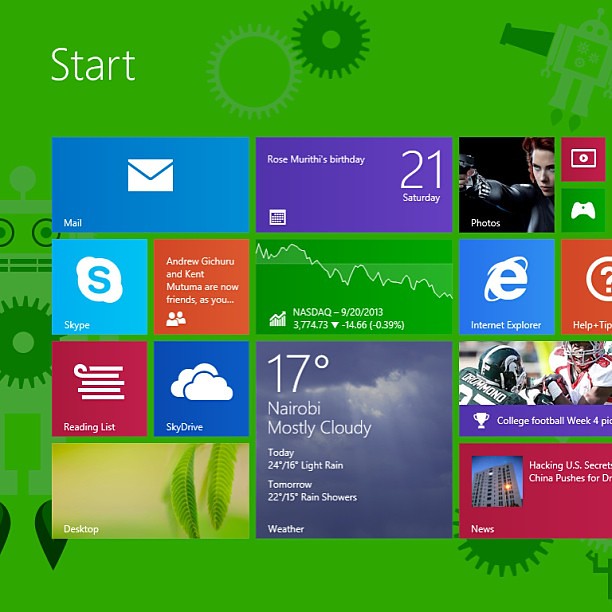Displayed on the computer screen is a green background featuring various functional widgets arranged neatly across the interface:

- **Top Left Corner:**
  - A blue rectangle labeled "Mail" with an icon of a white envelope.
  
- **Middle Section:**
  - A purple rectangle announcing "Rose Murphy's Birthday - 21 Saturday."
  
- **Right Section:**
  - An image of a woman holding a gun labeled "Photos."
  - An image with a play button and an Xbox controller icon.

- **Lower Section:**
  - Various icons including an image for Internet Explorer, a graphical representation of NASDAQ stock market data, and a Skype icon.
  - Additional icons for Reading List, SkyDrive, and Desktop.
  
- **Bottom Section:**
  - A weather widget displaying the current temperature in Nairobi as 17°C, mostly cloudy, with an expected range of 24°C/16°C and light rain for the day.
  - Forecast for the next day includes 22°C/15°C with rain showers.
  - The bottom of the widget is labeled "Weather."

Each element is clearly demarcated, providing a user-friendly interface for accessibility and information.